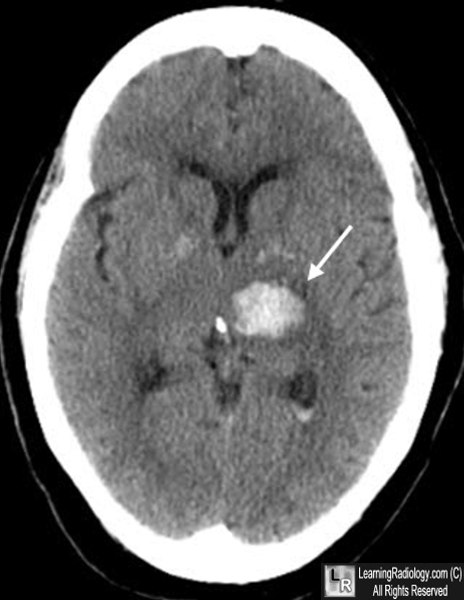This is a detailed image of a human brain captured through medical imaging, possibly an MRI or CT scan, viewed from above. The scan reveals the brain's dark gray matter surrounded by the bright white outline of the skull. Noteworthy is a large, white, circular mass situated near the center of the brain, slightly to the right, which is highlighted by a white arrow pointing directly at it. This mass stands out against the otherwise gray and uniform brain tissue, indicating a potential anomaly such as a tumor. The background of the image is uniformly black, contrasting sharply with the bright details of the skull and the highlighted area within the brain. At the bottom right corner of the image, there is a caption in white text reading "learningradiology.com, all rights reserved," signifying the source and copyright information.